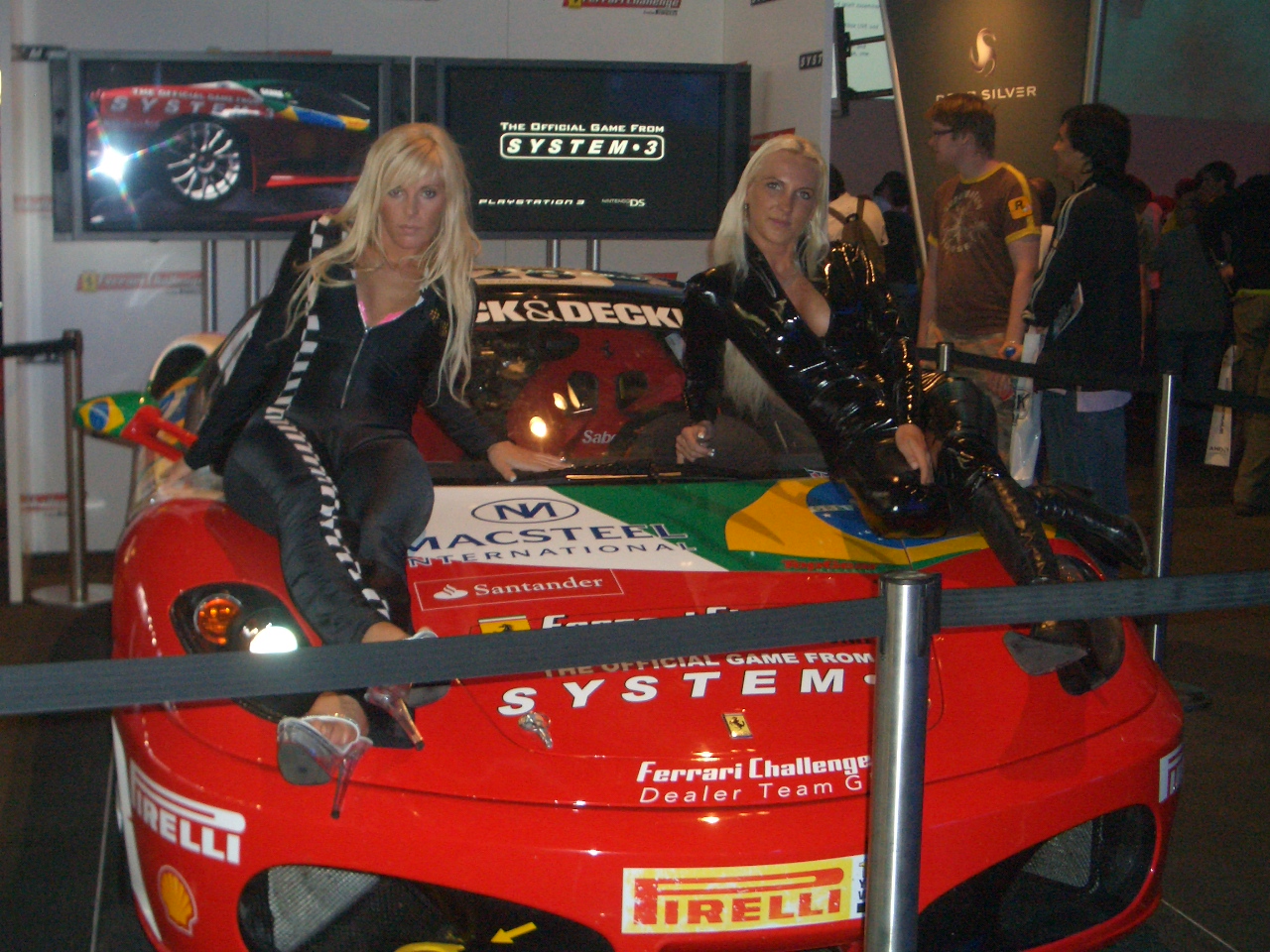In this indoor image, we see a roped-off display featuring a striking red Ferrari race car adorned with various logos in white, green, yellow, and blue. Notable logos include Ferrari Challenge, Pirelli, Max Steel, and Black & Decker, with "The Official Game from System 3" prominently displayed on a screen in the background. Two female models with long blonde hair are posing on the hood of the car, which is situated behind black ropes, suggesting an auto show setting. 

The model on the right side (from the driver's perspective) wears a form-fitting black outfit with racing check accents and high heels, while the model on the left dons a shiny, lycra spandex bodysuit and black boots. The left model leans on the windshield, staring directly at the camera as spectators and TV monitors populate the background. Both models exhibit a slightly bored expressions but maintain a professional demeanor, enhancing the allure of the display.